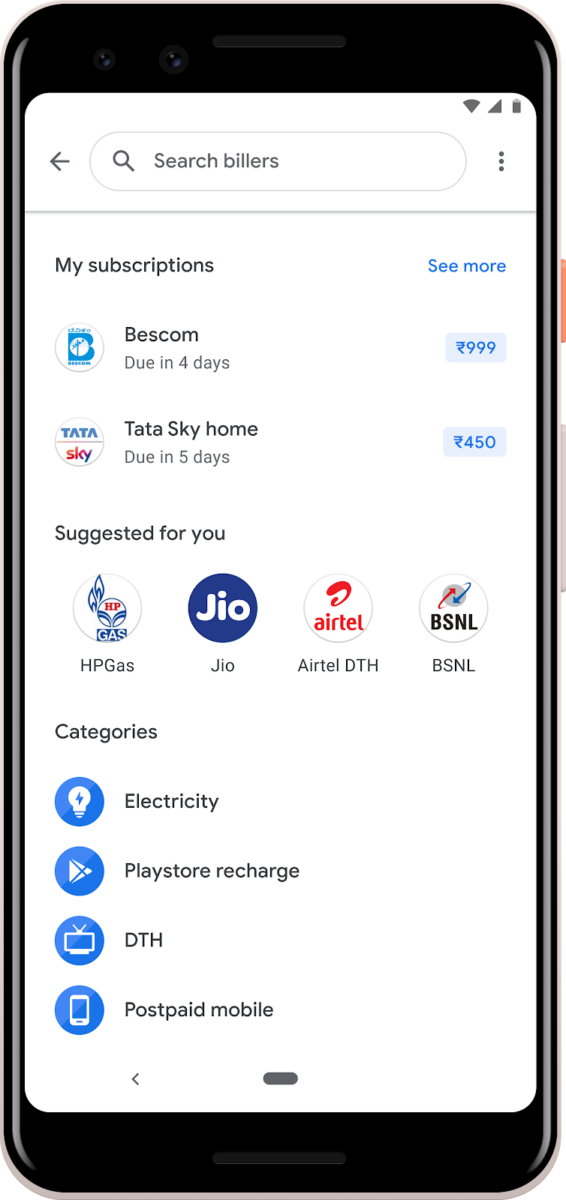This image captures a detailed screenshot of a smartphone's screen, which appears to be set against a blurred background, giving the illusion of a photograph of the phone itself. At the top of the screen, a web page is displayed with a prominent search bar labeled "Search Billers" and a small magnifying glass icon to the right. Adjacent to this, on the far upper right, are indicators for battery life, Wi-Fi connectivity, and signal strength.

Beneath the status indicators, the page header reads "My Subscriptions" followed by a clickable "See More" link highlighted in blue. In the subscription section, two entries are listed: "Best Calm" which is due in four days and costs $9.99, and "Tata Sky Home" due in five days, costing $4.50. Each subscription entry is accompanied by a small profile icon—one with a blue "B" for Best Calm and another that simply states "Tata Sky" for Tata Sky Home.

Following the subscriptions, a "Suggested for You" section lists potential services including HP Gas, Jio, Airtel, DTH, and BSNL. Below this section, the "Categories" heading introduces various service categories, each marked with blue icons: Electricity, PlayStore Recharge, DTH, and Postpaid Mobile. The overall layout and iconography suggest a well-organized bill management or service subscription application.